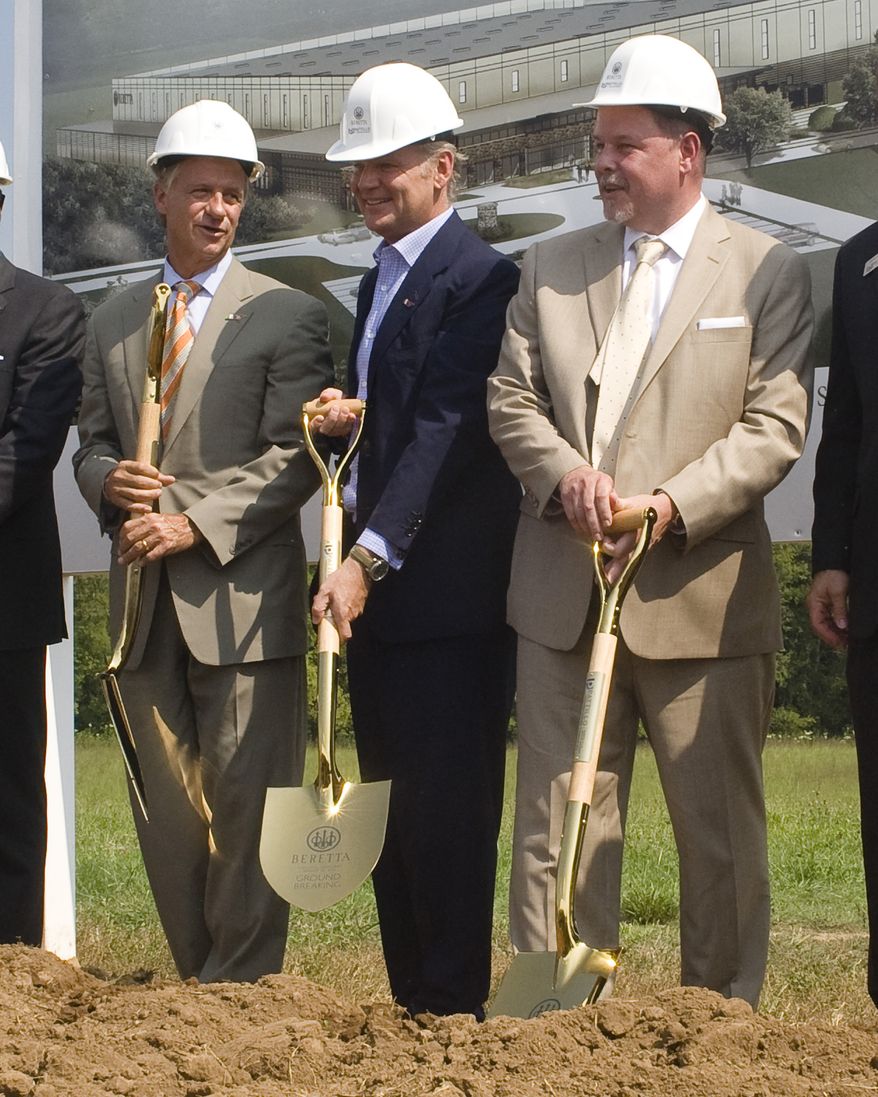The image captures three smiling, white-skinned CEOs or top-level managers from the group Beretta at a groundbreaking ceremony, signifying the start of a new factory construction. All three men are dressed in suits and wearing white hard hats, with the two on either side clad in tan suits and the one in the middle in a black suit. They are holding gold-plated shovels inscribed with the Beretta logo, which features three towers encircled within a ring. In the background, a mock-up of the future factory can be seen, indicating the planned construction site. While one CEO has already placed his shovel into the ground, the other two hold theirs upright. The scene takes place outside on a clear day, with a pile of dirt in front of them, ready for shoveling. A couple of additional men are partially visible but not the focus of the image.